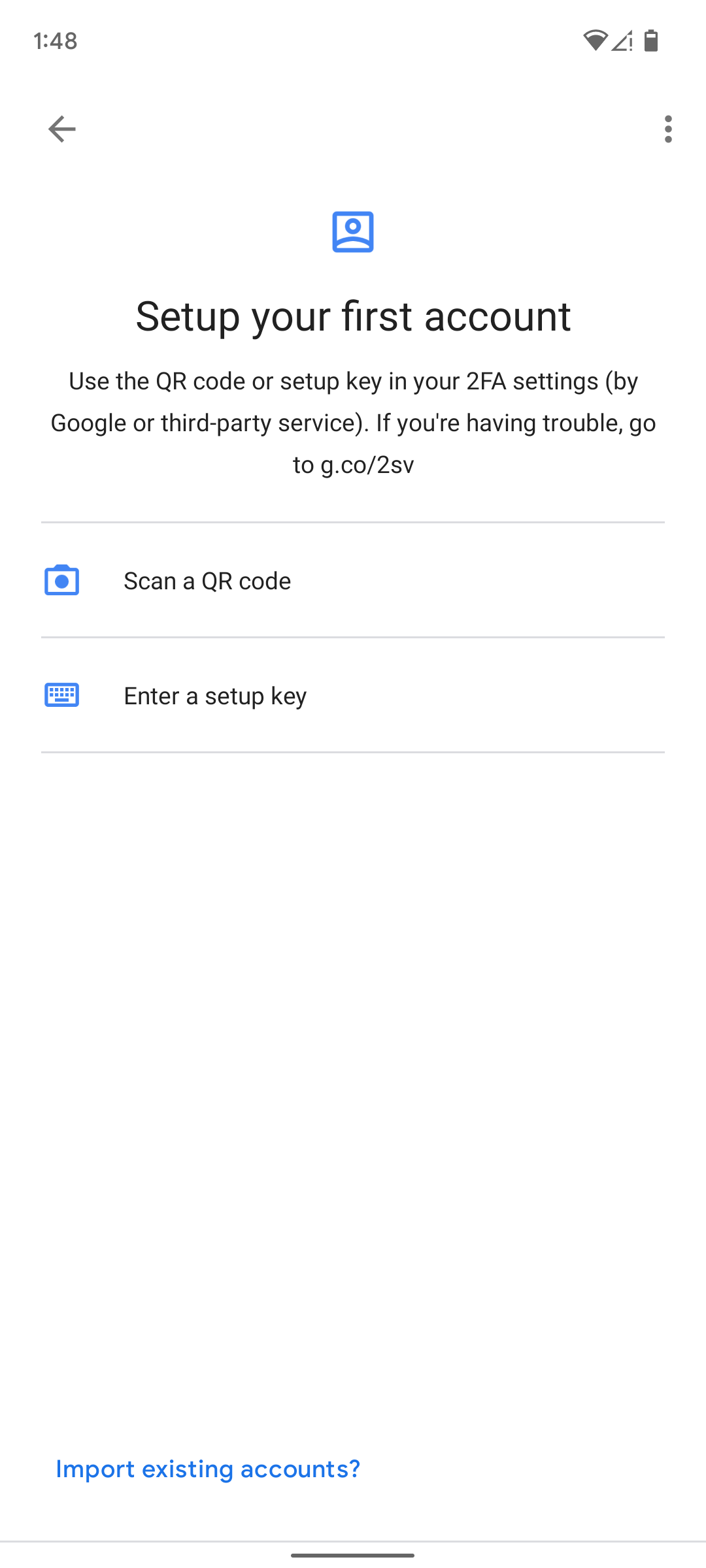The image is a mobile screenshot depicting an account setup page. The background is predominantly white. At the top left corner, the time is shown in a dark gray font, reading "1:48." On the top right side, there are several icons, including a Wi-Fi signal, a battery, and a triangular symbol. 

Directly beneath the time, a gray left-arrow button indicates navigation, while three vertical dots on the far right suggest a drop-down menu. The primary content of the screen features a centered blue icon resembling a generic profile picture, showing a circle for the head and shoulders.

Below this icon, bold black text commands attention, stating "Set up your first account." Underneath, smaller black text provides instructions: "Use the QR code or setup key in your 2FA settings (by Google or third-party service). If you're having trouble, go to g.co/2SV." 

A thin gray separator line follows, beneath which, on the left, a blue-outlined camera icon appears with the label "Scan a QR code" to its right in black text. Another thin gray separator line separates this section from the next, where a blue-outlined keyboard icon is seen on the left, labeled "Enter a setup key" in black text on the right. 

Following another thin gray separator line, there is ample blank white space. At the very bottom of the image, blue text reads "Import existing accounts," just above a final thin gray line marking the bottom edge of the screen.